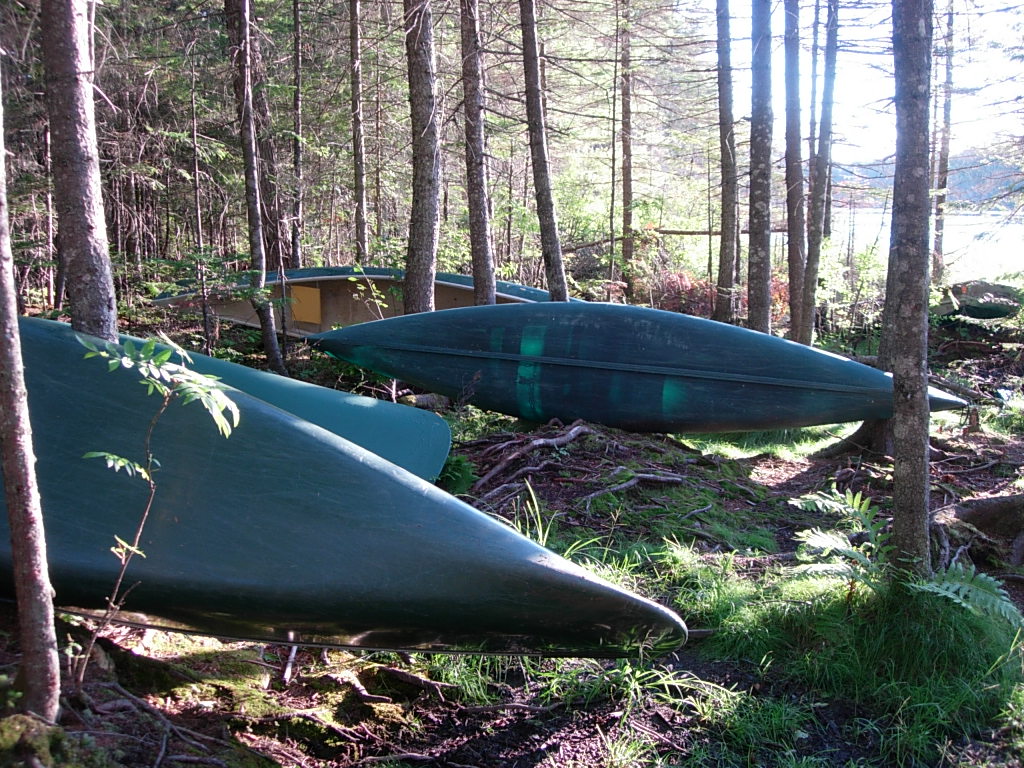In this detailed image of a forest, several emerald green canoes lie on the rough and irregular ground amongst an intricate web of tree roots, small grasses, and patches of moss. The forest features an understory adorned with ferns and tree trunks covered in lichen. Most of the trees, primarily hemlocks, display bare branches in the lower parts, with many small dead twigs, suggesting either a fall or winter season. In the foreground, a small sucker sapling stands just before one of the canoes. The upper right corner of the image reveals a brightly lit body of water, with light reflecting vividly, hinting at daylight hours. Beyond the water, there's a scenic view of mountains, completing the picturesque landscape. Scattered amidst the trees, one can see the interior of a canoe showing wooden material, and parts of potential rowing equipment peeking out.